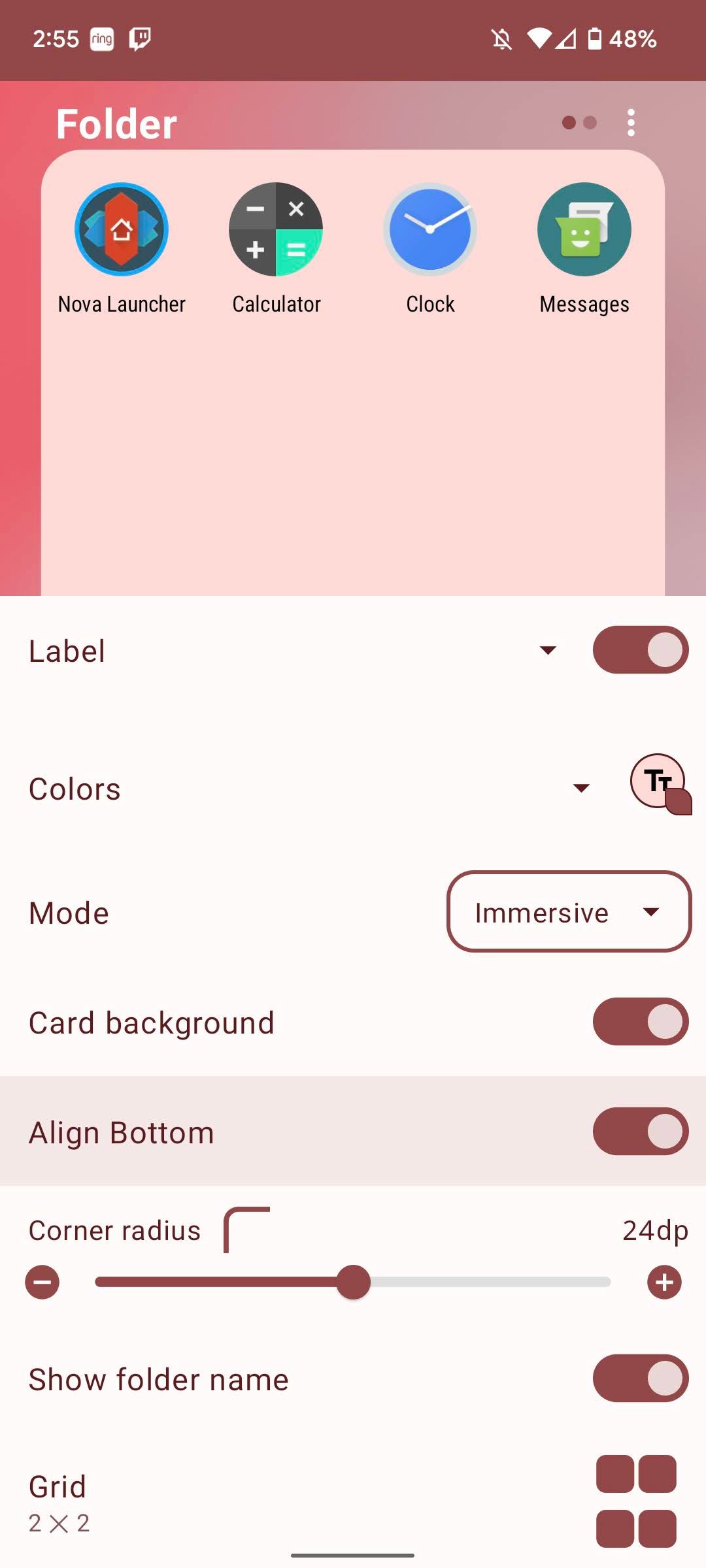A detailed screenshot of a smartphone interface displays the status bar at the top indicating the time as "2:55" with various status icons, alongside a battery indicator showing "48%". Below the status bar is a folder containing multiple app icons, including Nova Launcher, Calculator, Clock, and Messages. 

The interface further showcases customization options for the folder with labels such as "Colors" and "Mode", with "Immersive" selected. Additional settings include toggles for "Card Background", "Align Bottom", and "Corner Radius", which feature plus and minus buttons for adjustment. The option to display the "Folder Name" is also visible. There is a "Grid" setting currently set to "2x2", accompanied by a visual representation of this grid layout. All text and icons are presented in a burgundy-pink color on a soft pinkish-white background, creating a cohesive and aesthetically pleasing theme.